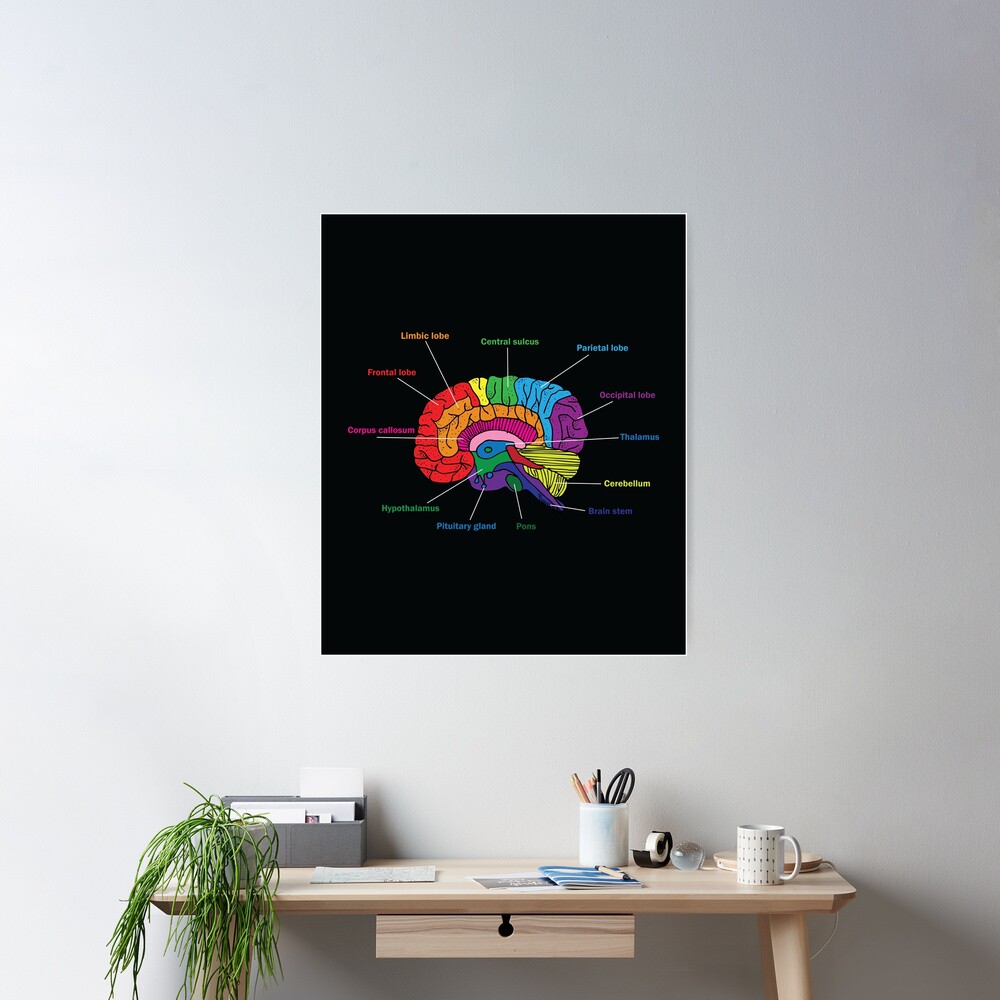The image showcases a compact, modern office setup centered around a light wood desk with a single black-knobbed drawer in the middle. On the desk's left side, an overgrown succulent and a small tray holding mail and various papers can be seen. The desk's center features an assortment of pamphlets and brochures, flanked by a white mug with polka dots, possibly containing liquid. Nearby, a cup holds pencils, scissors, and a tape measure, along with a roll of scotch tape. On the right side of the desk stands a minimalist, tall, thin white lamp. Above the desk on a white wall, a large black poster of an anatomical brain diagram is prominently displayed. The diagram vividly color-codes and labels different brain regions in bright, highly saturated colors like reds, oranges, purples, pinks, blues, yellows, and various shades of green and purple.